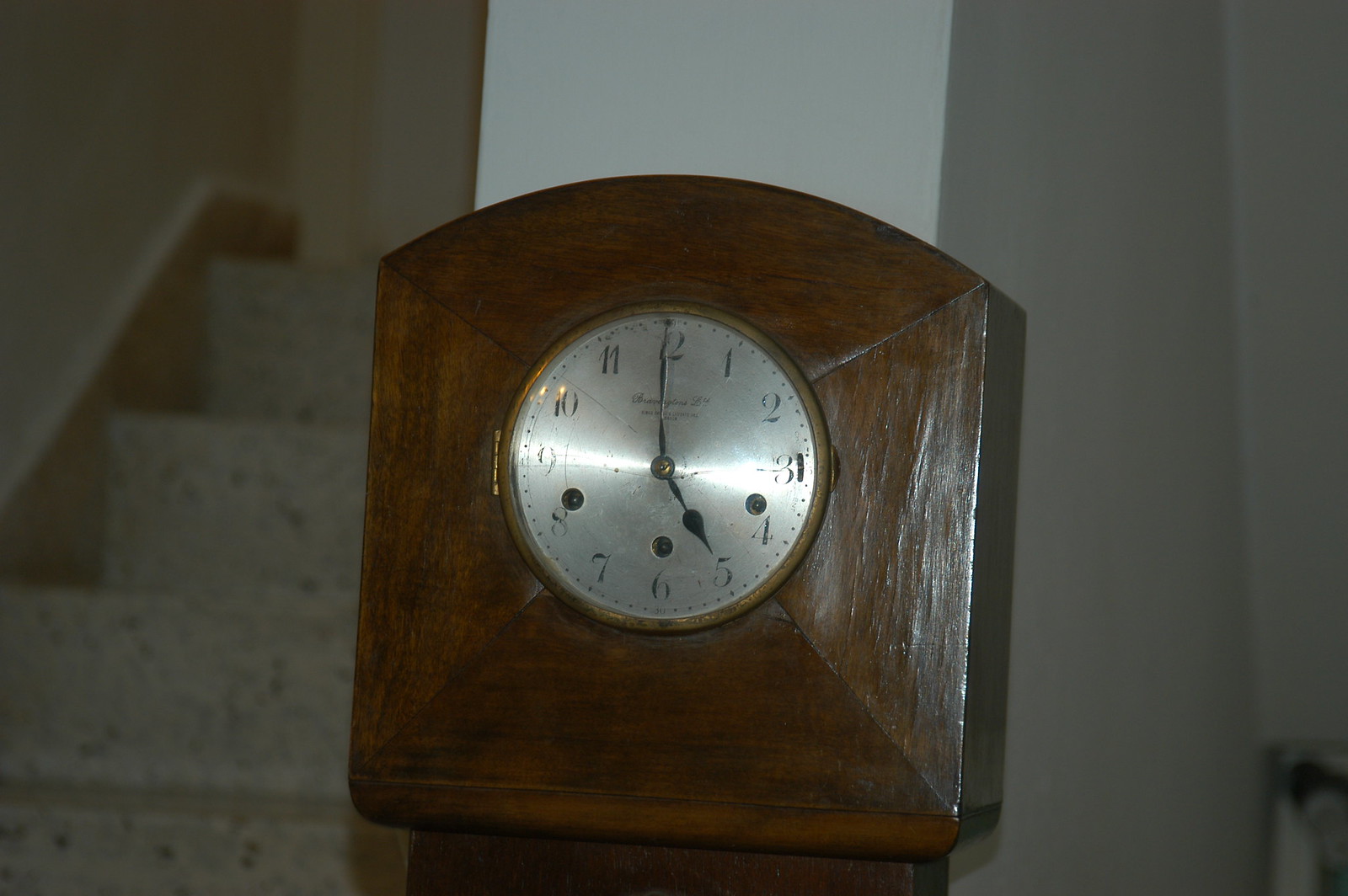In this dimly lit photograph, a wooden clock is prominently featured against a backdrop of white walls. To the left of the clock, a set of stairs made from a speckled material ascends, adding texture to the scene. The clock, which is square-shaped with an arched top, showcases a round, silver face. The hour and minute hands are black with teardrop-shaped tips. Black numerals mark the hours, while small black dots indicate the minutes, with more pronounced black lines denoting the five-minute intervals.